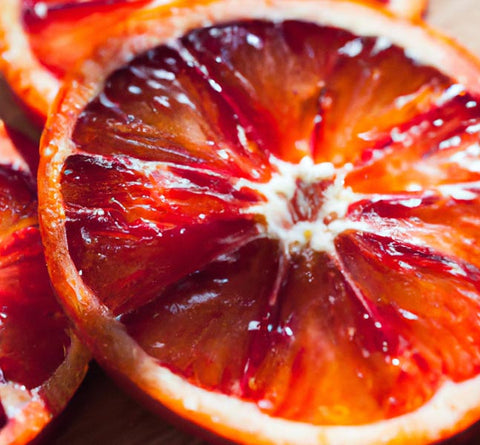This detailed, close-up photograph captures a freshly cut blood orange in an artsy and professional manner. The primary subject is a prominently placed circular slice in the foreground, which showcases its vibrant red and fiery orange hues, appearing wet and juicy as if it was just cut. The orange's segmented interior glistens, with visible pulp and a pit in the middle, emphasizing its fresh and ripe quality. Surrounding this central slice, additional slices are layered in the background, creating a stacked effect that hints at more fruit beyond the immediate focus. The outer rim of the orange is a bright orange, contrasting beautifully with the richly red segments inside. Subtle shadows and natural lighting, possibly coming from the upper right, add depth and dimension to the image, highlighting the texture and juiciness of the fruit. The backdrop is ambiguous, potentially a wooden surface, but it's minimal enough to keep the attention firmly on the sumptuous and inviting blood oranges.